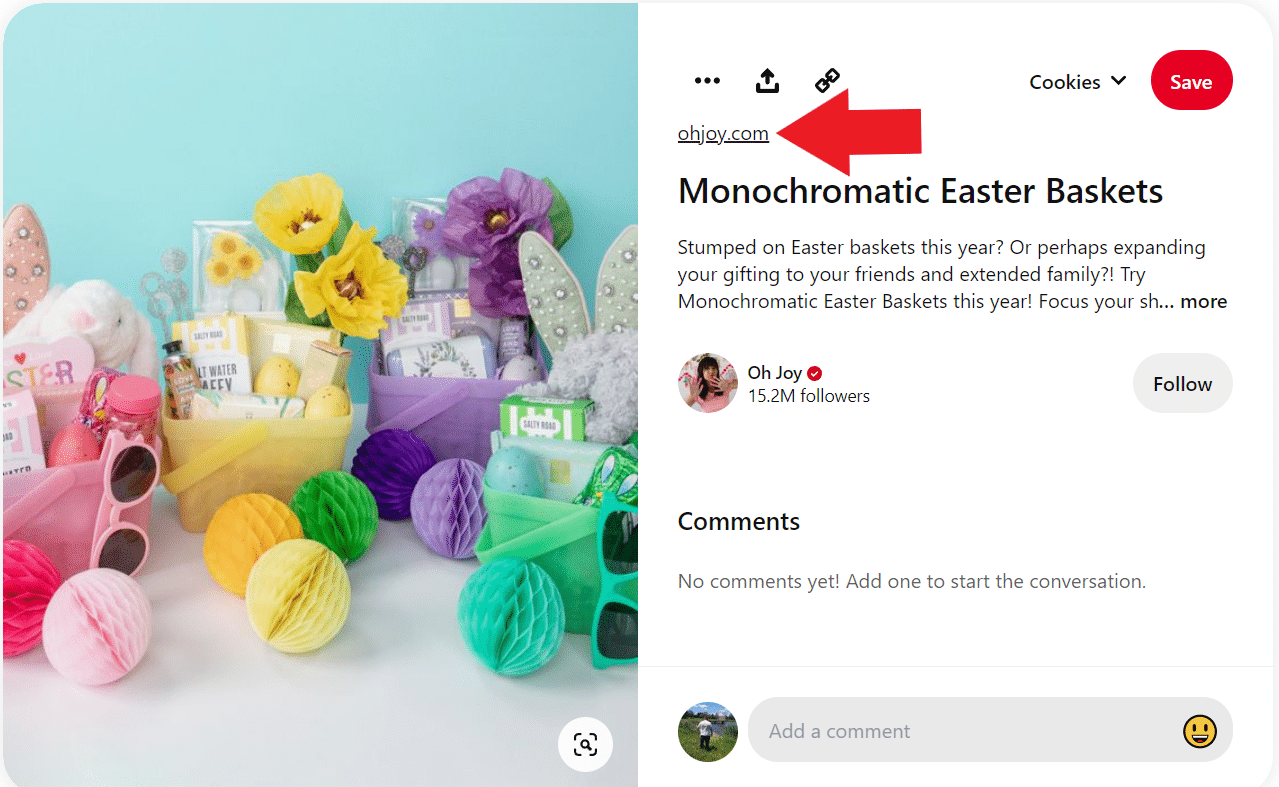The image showcases a webpage from OldJoy.com, highlighted with a large, prominent red arrow that directs viewers to the site. At the top-right corner of the webpage, there are three vertical dots indicating a dropdown menu, alongside icons for uploading, linking, and cookie options. A “Save” button is also displayed within a distinct red oval.

Centered on the page, a bold header reads "Monochromatic Easter Baskets," inviting users to explore ideas for creating themed Easter gifts. The subtitle questions: "Stumped on Easter baskets this year? Or perhaps expanding your gifting to your friends and extended family?" It then suggests trying monochromatic Easter baskets and teases additional content with a "read more" option.

The page highlights OldJoy.com, a popular website with 15.2 million followers, known for selling creatively themed Easter baskets. Each basket is curated to match a specific color. For instance, a pink basket contains pink-rimmed sunglasses, pink-wrapped Easter eggs, and jars of pink sweets. A yellow basket features yellow flowers, yellow-wrapped Easter eggs, and various yellow blooms like daisies and sunflowers. Additional ready-made baskets come in colors like purple, lilac, and mint green, each meticulously filled with color-coordinated Easter-themed items.